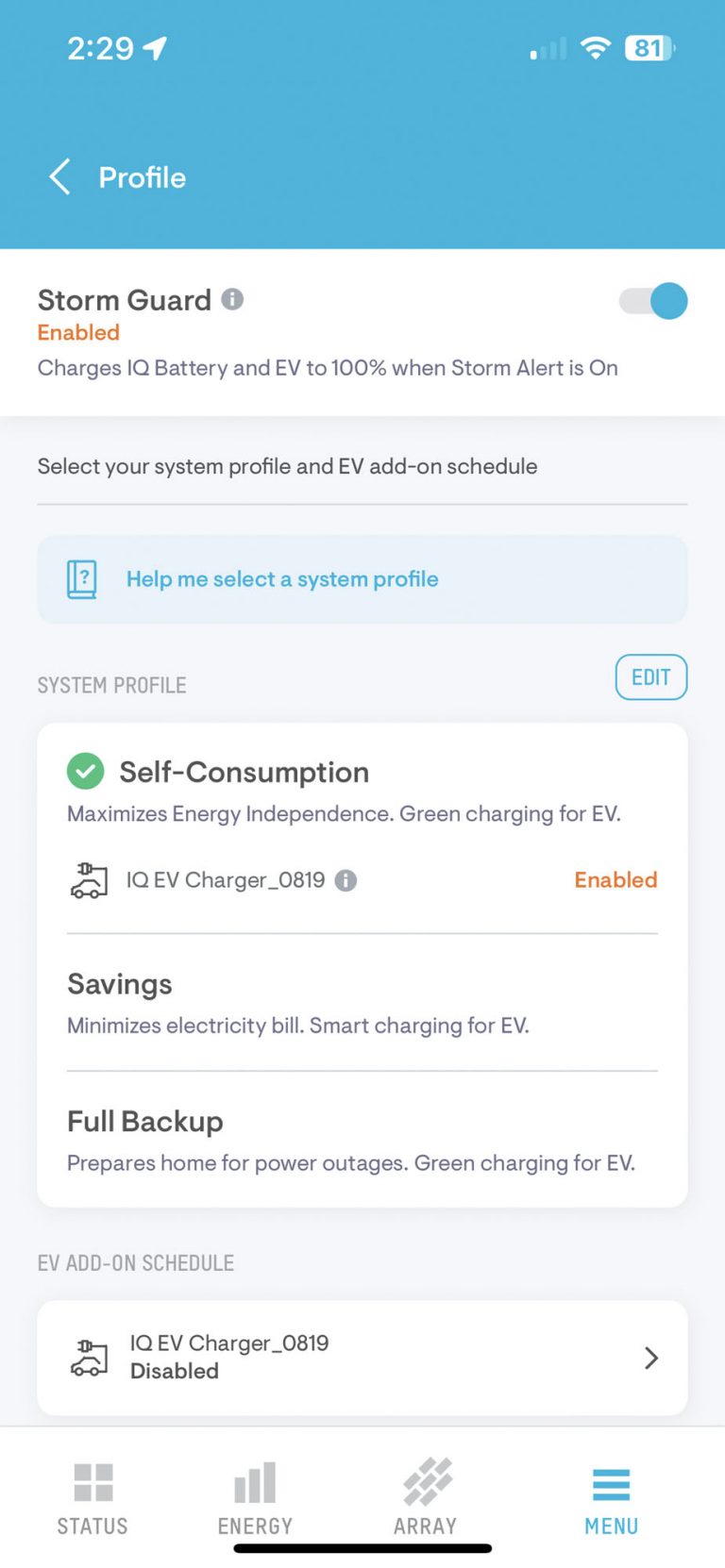The image is a mobile screenshot detailing various settings for a feature called "Storm Guard." At the top of the screen, a blue rectangle displays the current time as 2:29 and shows the battery at 81% charge. To the left, there is a "Profile" option with an accompanying arrow. Below this, in a white bubble, the title "Storm Guard" is displayed alongside an enabled toggle switch. This feature, when activated, charges the IQ battery and an electric vehicle (EV) to 100% whenever a Storm Alert is issued.

Beneath this section, a gray box presents additional options. These include "Select Your System Profile" and "EV Add-On Schedule." A blue bubble labeled "Help Me Select a System Profile" is also present for user assistance. Further down, the current System Profile is shown with an "Edit" button to the right. The profile selected is "Self-Consumption," highlighted with a green checkmark and a brief description, "Maximizes energy independence."

The next item on the list is "Screen Charging for EV," which pertains to an "IQ EV Charger_0819" and shows that the setting is enabled. This section features a small icon of a car being plugged in. Following this is a "Savings" option aimed at minimizing electricity bills through smart charging for the EV. Further down, the "Full Backup" option prepares the home for power outages while providing green charging for the EV. The "EV Add-On Schedule" is mentioned again in a white bubble, where the "IQ EV Charger_0819" appears as disabled, accompanied by the same car icon.

At the bottom of the screenshot, additional menu options are visible: "Status," "Energy," "Array," and "Menu," with the "Menu" option highlighted in blue.